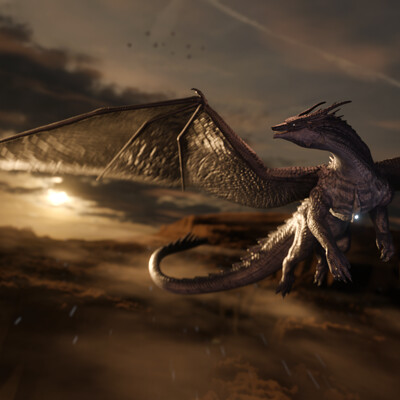The image is a highly detailed 3D render of a sci-fi-inspired dragon flying in a hazy, brown-tinged sky with the sun partially obscured by dark clouds. The dragon, rendered in a dark brown, almost shiny and reflective texture, features a long, curly tail, two large bat-like wings, and four limbs. It has a thick neck and a face more reminiscent of a lizard than a traditional dragon, accented by two backward-pointing horns. The creature's posture is peculiar; its head is twisted back towards the sun, its legs are dangling as if walking, and a bright, blue LED light illuminates from a plate on its chest. Beneath the dragon, the faint outline of a brownish terrain can be seen, adding a grounded element to the otherwise fantastical scene.